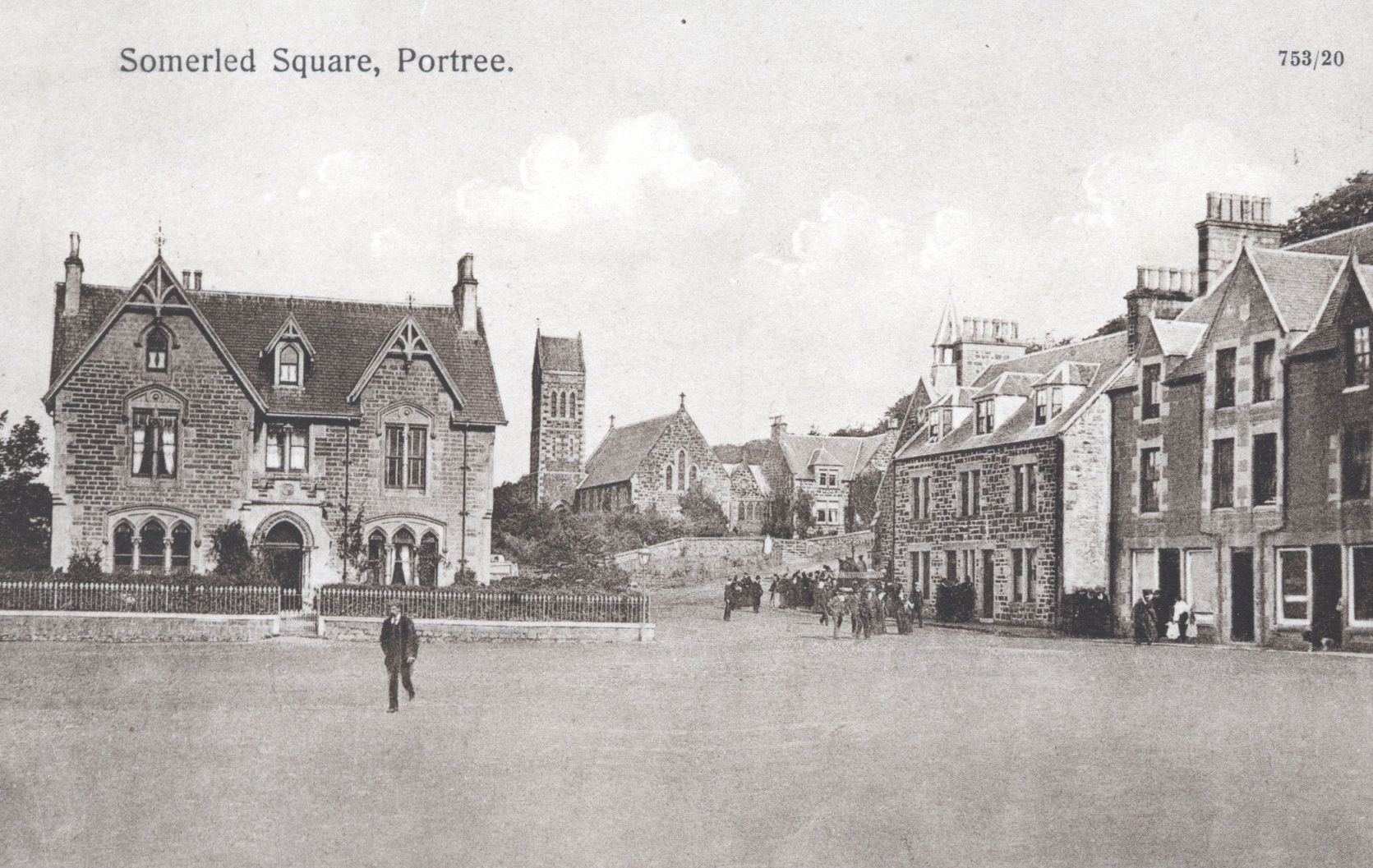The image is a black-and-white photograph identified as Somerled Square in Portree, with the text "753/20" in the top right corner. The scene captures an expansive courtyard in the foreground, leading to a road that vanishes into the distance. On either side of the road, there's a collection of heavy, multi-story brick buildings, possibly old mansions or churches, characterized by chimneys and towers protruding from their roofs, some adorned with wood trim. One prominent building to the left boasts two stories and an attic, along with a dark, slanted roof and chimneys on both sides. To the right, similar-height buildings feature slanted awnings. The far distance reveals a large, church-like structure with a noticeable steeple. People are scattered throughout the scene, some walking in the courtyard, others riding horses and carriages on the road, providing a glimpse into the bustling activity of the square. The sky above is dotted with white clouds, completing the historic and lively atmosphere of Somerled Square.